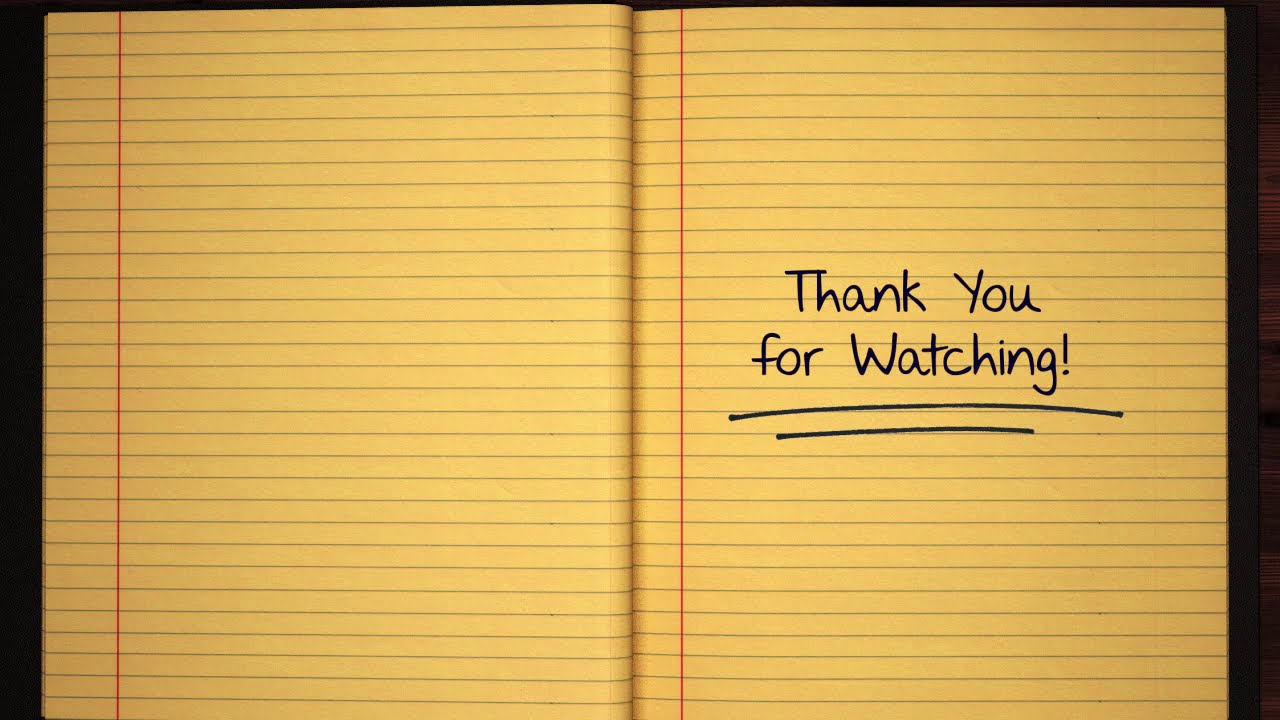This digitally altered image depicts an open, yellow-hued, college-lined notebook with black borders, set against a rich mahogany wooden background. The notebook's pages are lined with horizontal blue lines and feature a vertical red ledger line on the left. In the middle of the right page, the handwritten text, "Thank you for watching!" is prominently displayed and underlined twice. The text appears to have been added digitally, enhancing the manipulated and computer-generated appearance of the overall image.